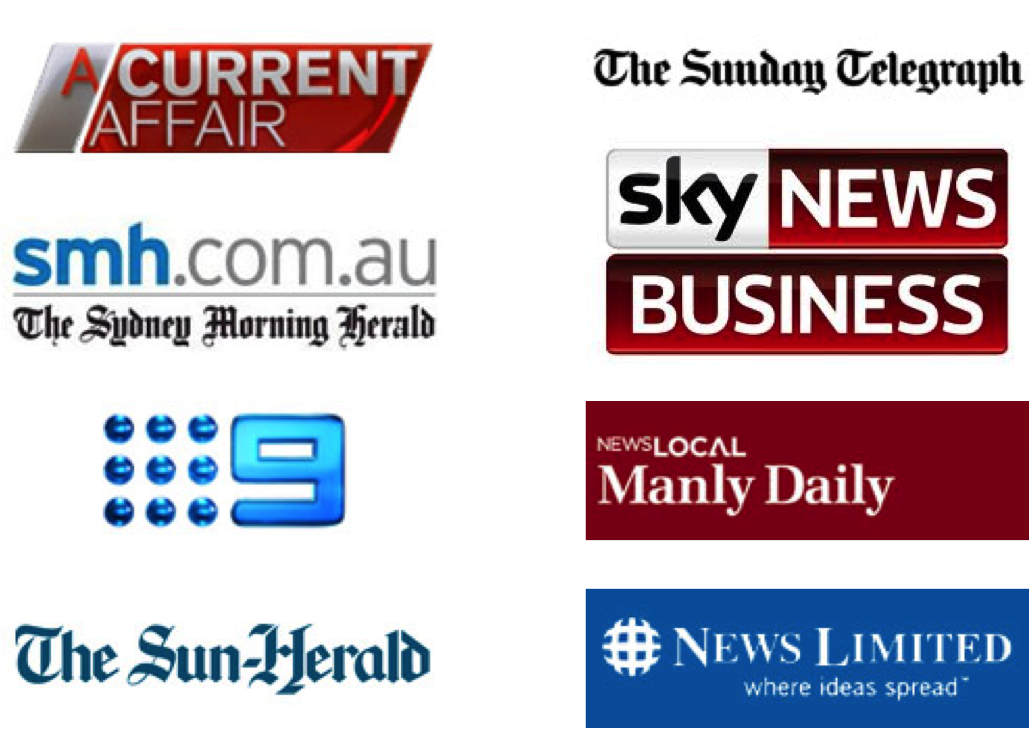Screen capture of a media listing on an all-white background, featuring two columns and four rows.

**Top Left:**
- **Current Affair**
  - Displayed on a parallelogram with a slanted right side.
  - Predominantly red (85%), with a small white section on the left.
  - "A Current" is in bold white font under "Affair," which is in a different font style.

**Top Right:**
- **The Sunday Telegraph**
  - Written in bold black font with a medieval script style.

**Second Row Left:**
- **smh.com.au**
  - The Sydney Morning Herald's website.
  - "SMH" is in blue, while ".com.au" is in gray.
  - "Sydney Morning Herald" is written in bold black, medieval-style font.

**Second Row Right:**
- **Sky News Business**
  - Displayed on two separate banners.
  - "Sky" on a white background with black text.
  - "News Business" in all caps, white text on a black-to-red gradient background.

**Third Row Left:**
- **Nine Dots**
  - "Nine" written next to nine blue dots, all in blue.

**Third Row Right:**
- **News Local, Manly Daily**
  - Both phrases in white text on a burgundy background.

**Bottom Left:**
- **The Sun Herald**
  - Displayed in medium blue with medieval font style.

**Bottom Right:**
- **News Limited**
  - Logo featuring a globe with lines crossing it vertically and horizontally.
  - White lettering on a blue background with the tagline "where ideas spread."